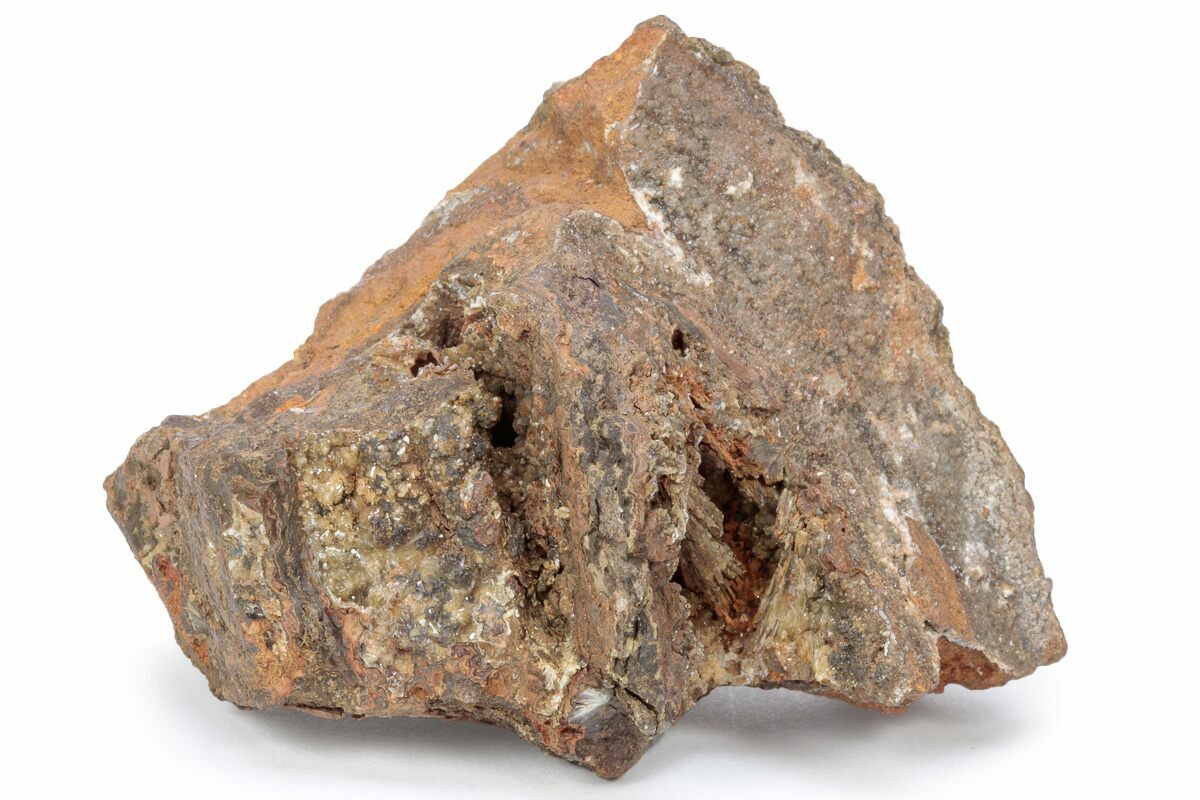The image features a single, notably large rock positioned against a stark white background, indicative of a professional photo shoot. The rock boasts a jagged and somewhat triangular shape, with its right side appearing larger than the left. Its coloration is predominantly a mix of gray and terracotta, with the terracotta hue most prominent on the top. Intermingled throughout the rock are streaks of pale orange and white specks. The front surface is adorned with gold-speckled cracks, adding to its intricate appearance. Additionally, the rock displays large holes and crevices, suggesting a natural history of erosion or an aquatic environment, with smaller lumps clinging to its surface, reminiscent of marine life attachment. White vein-like materials encircle parts of the rock, further hinting at possible petrification or mineral deposits accrued over time.